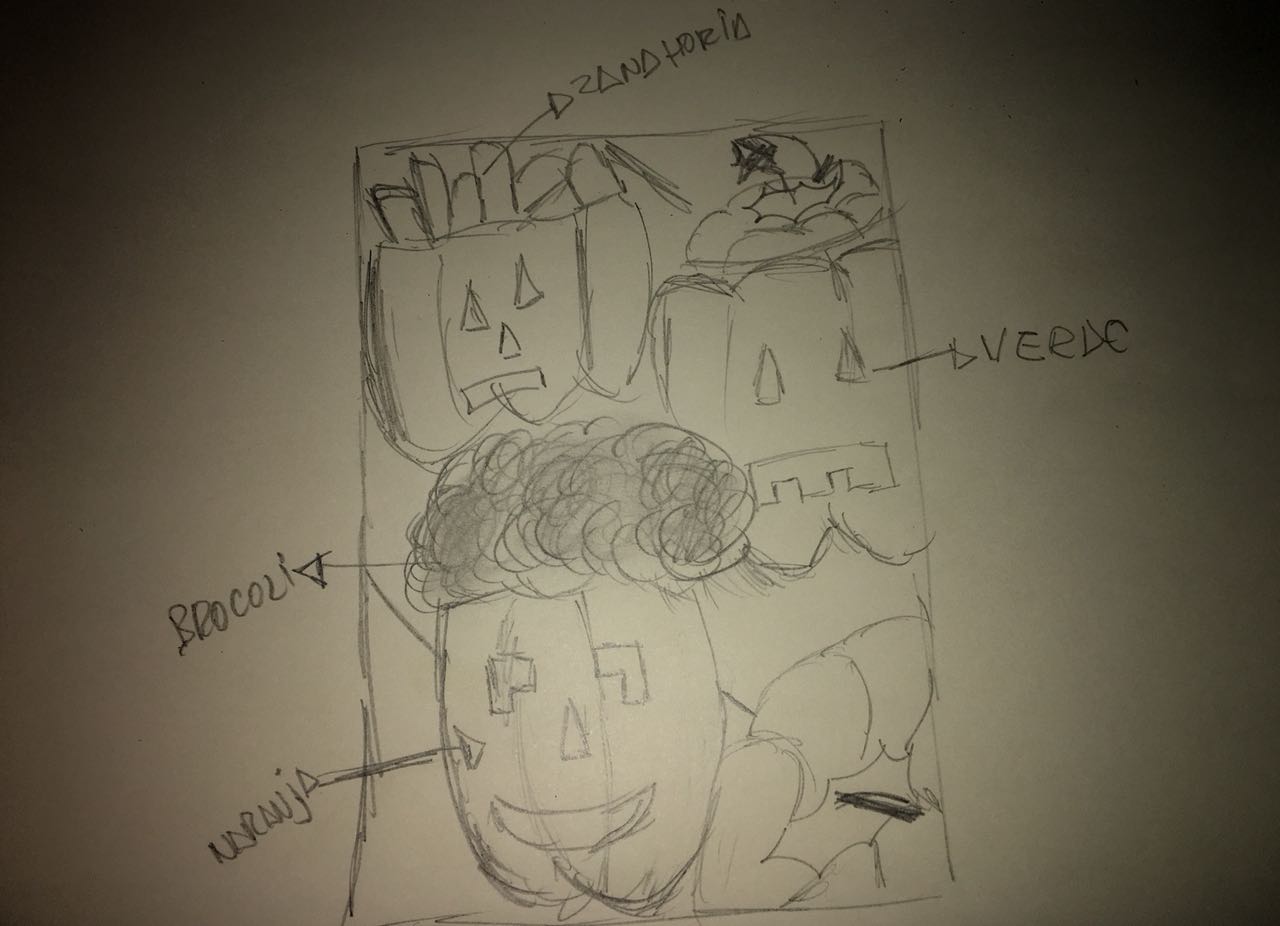The image features three intricately sketched jack-o'-lanterns, each with distinctive characteristics. The first jack-o'-lantern, positioned in the top left corner, is adorned with what appears to be hair. Notably, the word "Zanahoria," which means carrot in Spanish, is etched into its head with A's resembling triangles. 

The second jack-o'-lantern, situated to the right, has an unidentified object on its top that is suggestive of various shapes, potentially resembling French fries. This pumpkin bears the word "Vierde," which, although misspelled, could be intended to mean "verde" (green) in Spanish. 

The final jack-o'-lantern is positioned towards the front and features intricate details that make its crown appear like broccoli. It is labeled "broccoli" on its head. Additionally, the body of this pumpkin is marked with the word "Naranja," translating to orange in Spanish.

In the background, there is another jack-o'-lantern, partially obscured, making its facial details indistinguishable. Together, these elements create a whimsical scene, perhaps depicting a planned jack-o'-lantern party with a focus on colorful, vegetable-themed characters.